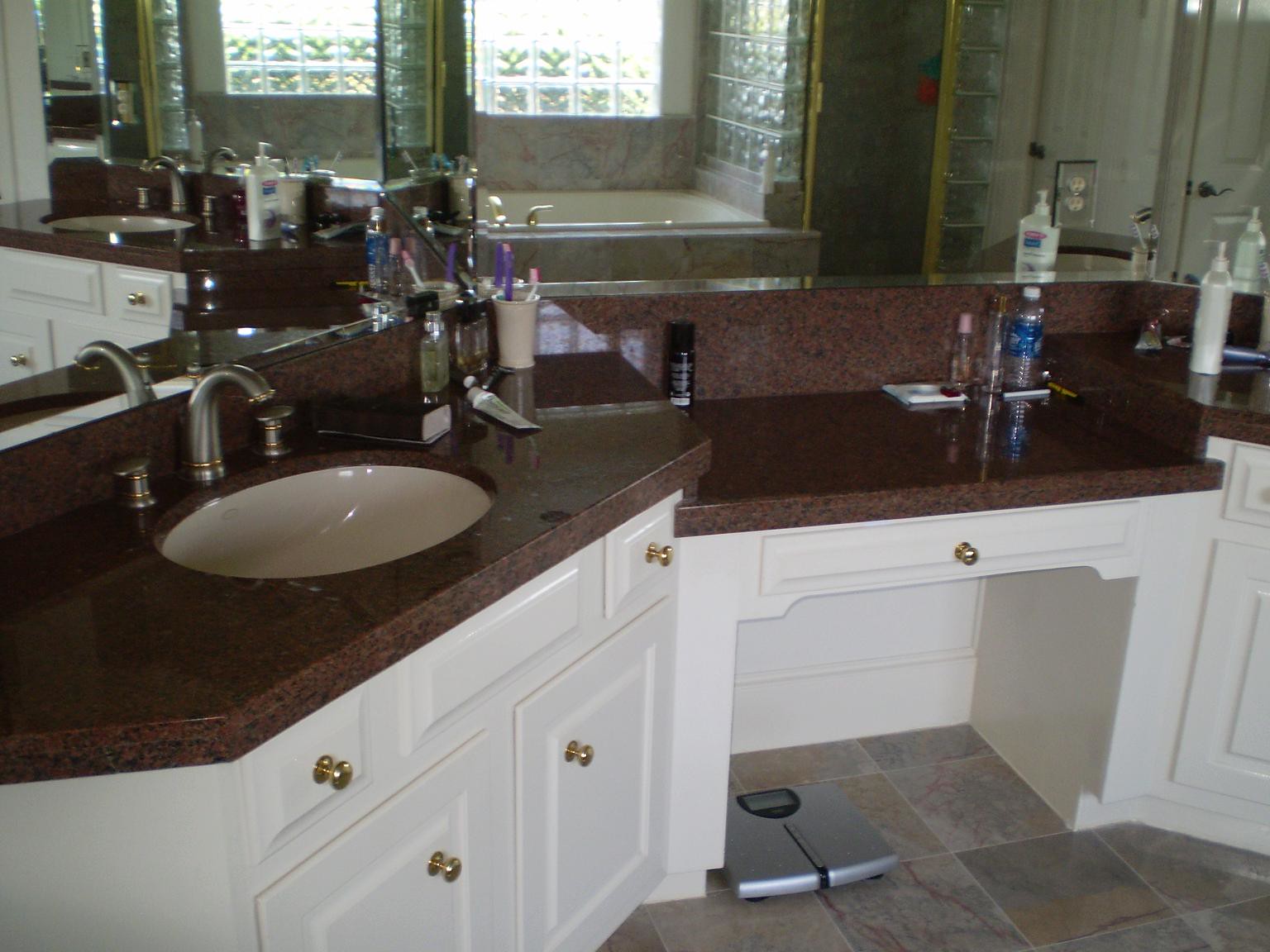This photograph captures the interior of a spacious bathroom, notably larger than typical residential bathrooms. It features a dual-sink setup with a vanity area in between. The countertop is a rich, dark granite, characterized by a reddish-brown base adorned with black speckles. The sink faucets are a blend of pewter and gold, adding a touch of elegance to the space. 

The flooring is composed of slate tiles in gray with subtle reddish hues. The vanity itself is painted white, complemented by gold knobs on the drawers and cabinet doors beneath. The countertop is cluttered with various items: square glass bottles, one with a black cap and another with a pump dispenser, a beige toothbrush holder, a water bottle, and a spray bottle. Additionally, there is a prominently displayed, mostly full, clear bottle of lotion.

This detailed arrangement of elements and finishes highlights both the functionality and the aesthetic appeal of this meticulously designed bathroom.